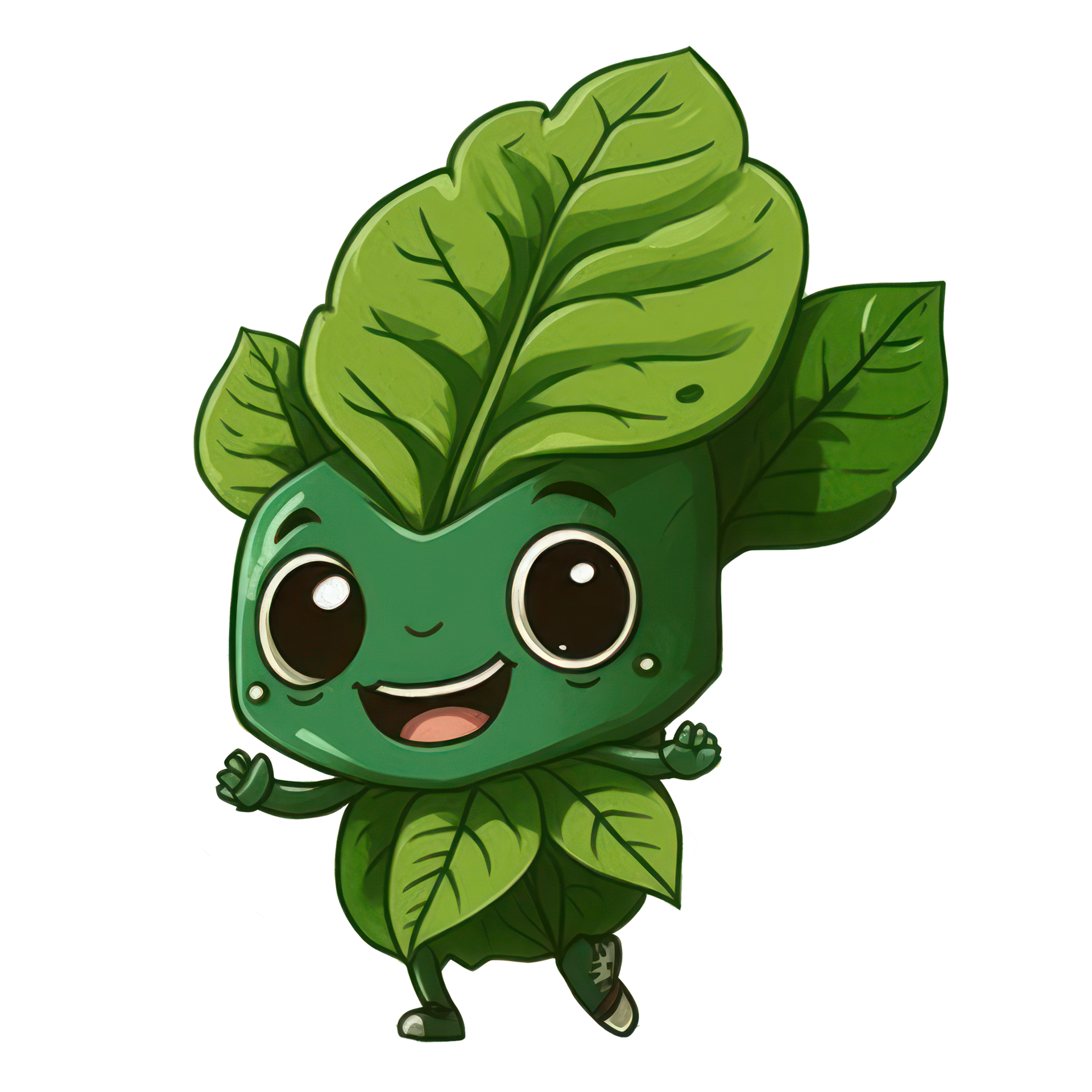This image depicts a highly animated and cheerful green cartoon vegetable character against a solid white background. The character features a large, veined leaf atop its head with two smaller leaves on either side, and a thin green stem. Its V-shaped head, with a green foliage body resembling a head of cabbage or lettuce, forms a large, almost brussel sprout-like figure. The character's facial expression is lively and joyful, with oversized black eyes, small eyebrows, a tiny nose, and a wide-open mouth revealing a pink tongue and a line of white teeth. It has small leaf-like fingers, and its right leg appears larger than the left. This leafy character is wearing green sneakers, holds its fists up as though cheering, and has two white dimples on its cheeks, along with two small bolt-like dots near its mouth. One of the top large leaves even has a distinct hole, adding to the character's detailed and intricate design.